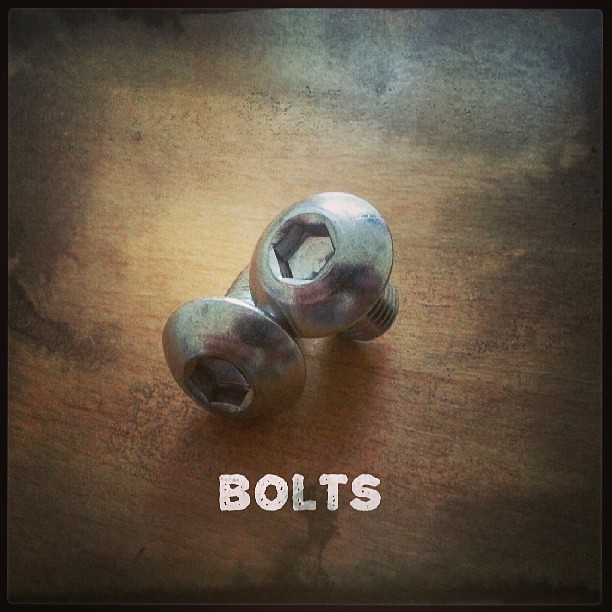The image presents an evocative close-up of two metallic bolts side-by-side, each with a hollow hexagonal head and a short thread. These shiny steel bolts are set against a rustic, dark wooden table that has scattered black specks, adding a rich texture to the backdrop. The lighting illuminates the bolts prominently, casting the surrounding areas into shadow, creating a striking contrast. The composition exudes a painterly quality, making the bolts appear almost like hand-rendered art rather than mere photographic subjects. At the bottom center of the image, the word "BOLTS" is displayed in bold white capital letters, grounding the metallic subjects with a defined title. Overall, the picture's artistic rendering and meticulous detail could easily make it a compelling piece of wall art.